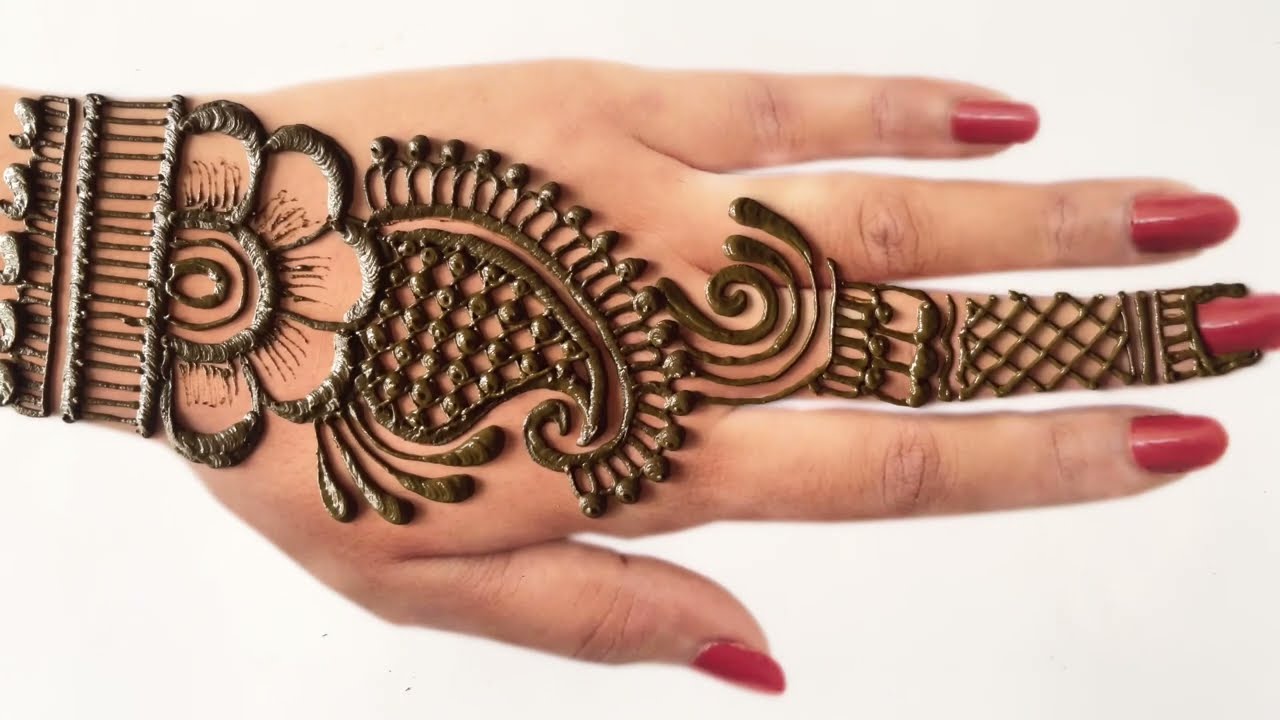The photograph features a pale woman's left hand with a tan undertone, laid flat against a white background. Her long nails are painted a vibrant red. The hand is adorned with an intricate and ornate henna design that is raised, appearing much like puffy or foaming paint in a deep brown color, indicating the henna is still drying. The design begins at her wrist, resembling a bangle, and extends onto the back of her hand where it features a large, elaborate flower. Above the flower, there is a seashell shape with leaf-like extensions and decorative beading, along with swirly lines. The intricate pattern continues with criss-cross lines traveling up the middle finger until reaching the nail. This finger has additional horizontal lines, while the henna on the other fingers is minimal, with just a small part extending to the index finger. The overall appearance of the henna showcases a detailed and ornate pattern still hardening on the skin.